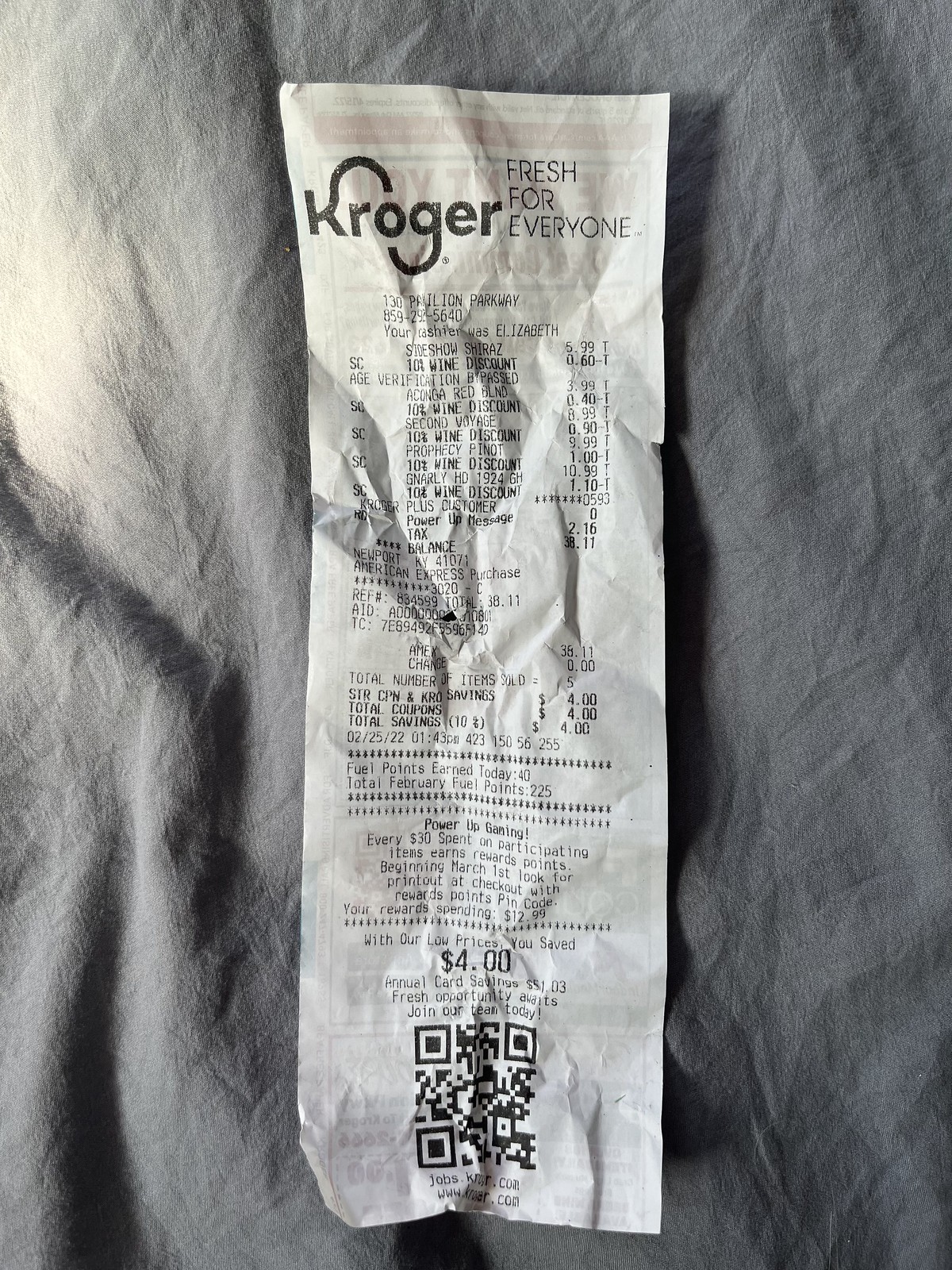This image features a crinkled, white Kroger receipt laid out on a similarly gray and crinkled sheet. The receipt prominently displays the Kroger slogan "Fresh for Everyone" at the top. It provides the store's address, 130 Pavilion Parkway, Newport, Kentucky, and a contact number, though it's partially obscured. The cashier’s name is Elizabeth. The receipt details that a 10% discount was applied to multiple wine purchases, resulting in savings of about a dollar or slightly more per bottle. The total balance due was $38.11, paid using an American Express card. There are $4 in savings highlighted in bold and an indication that 40 fuel points were earned from this transaction, bringing the total for February to 225 points. At the bottom, the receipt mentions a "Power-Up" event aimed at encouraging further purchases, includes a QR code, and references additional promotional details. The receipt lists a total of five items bought, with one of the listed items being alcohol amounting to $12.16.